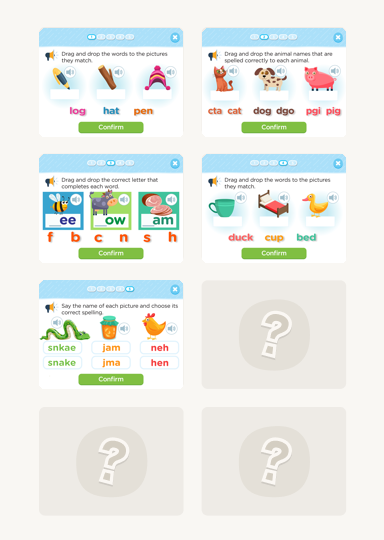The vertically rectangular image showcases a light tan background, partitioned into two main columns, each appearing as screenshots from a children's activity app. Both columns are divided into four blocks. The left column features three vivid images of a children's game, with the bottom block grayed out and marked by a question mark. The right column exhibits a similar layout, with its top two blocks containing game images and the bottom two blocks displaying gray question marks.

At the top left corner of the image, an instructional text reads, "Drag and drop the words so to the pictures they match." Below this directive, the game displays three images: a pen, a log, and a hat. Beneath these visuals, the corresponding words "log," "hat," and "pen" are listed, accompanied by a confirm button.

The other images within the columns also feature similar interactive activities, each culminating with a confirm button, but showcasing different sets of images for the matching game.